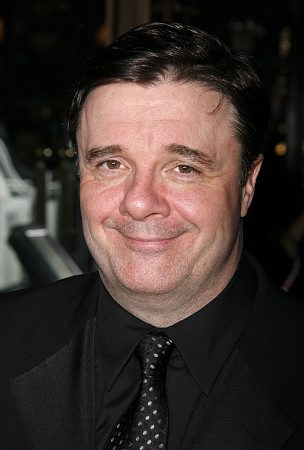This photograph showcases a middle-aged man, approximately 50 years old, with short, curly black hair. He is smiling warmly and looking directly into the camera. His attire consists entirely of black, including a black shirt paired with a black tie adorned with white dots. The background is completely blurry, making it difficult to discern any specific details behind him. The lighting is softened by the use of flash, which illuminates his face evenly without being too harsh, while the background remains significantly darker. The man bears a striking resemblance to Sean Astin.